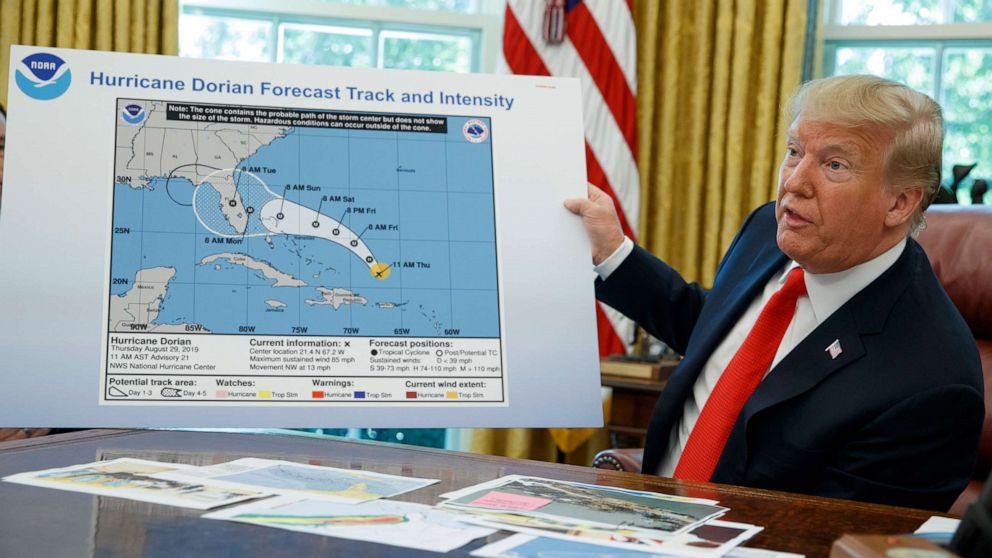In this high-quality photograph taken inside the Oval Office, President Donald Trump is seated at his large wooden desk, distinguished by its papers and photographs. Trump wears a dark navy blue or black suit, accented by a white collared shirt, a red tie, and an American flag pin on his lapel. He is seated in a red or maroon chair, with the room's classic yellow curtains and the American flag visible behind him. Holding the attention of the room, Trump raises a large placard with one hand. The top of the placard prominently reads, "Hurricane Dorian Forecast Track and Intensity," and displays detailed radar images from NOAA, depicting the storm's path toward Florida from August 29, 2019. The graphic includes nuanced details such as current information, forecast positions, and areas under watch or warning, with labels stretching from 11 a.m. Thursday to 8 a.m. Tuesday. Trump appears engaged, possibly speaking to someone off-camera, his mouth slightly open as he talks.